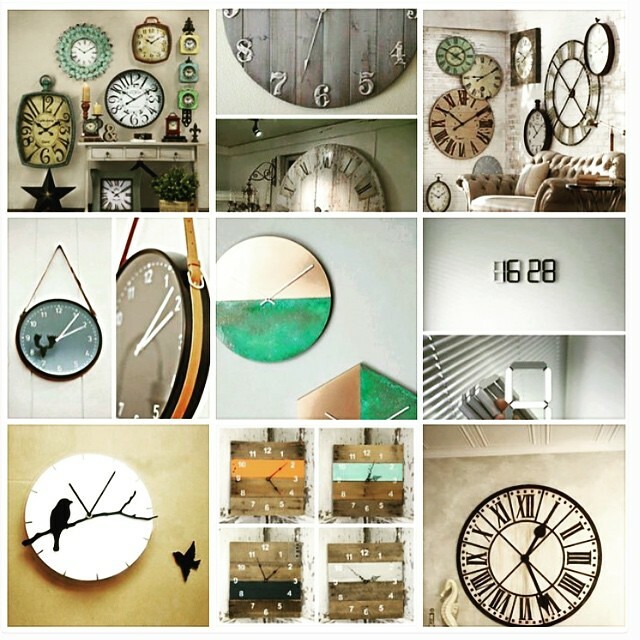The image is a detailed square collage featuring nine individual blocks, each showcasing a distinctive style of wall clock arranged in a 3 by 3 grid pattern. Each clock is uniquely designed, creating a harmonious yet varied tapestry of timepieces.

Starting from the top left, the first block displays a collection of analog clocks with different faces and frames in shades of teal, black, and light yellow. These clocks vary in shape, including squares and circles, and are all hanging on a wall. The second block is split horizontally, featuring Roman numerals on the bottom and numerical digits on the top. The right-hand side presents a series of round clocks of various sizes, including one peculiar clock set within a square frame.

The middle row left block shows identical clock images, divided in half and hanging by a tethered rope, exuding a rustic charm with gold and verdigris tones. The center block features two clock faces devoid of numbers, embracing minimalistic elegance with metallic and verdigris finishes. The middle right block displays a digital clock, uniquely designed to resemble wood with LED-style numbers.

In the bottom row, the leftmost block is home to a white circular clock featuring a black silhouette of a bird perched on a branch, absent of numerical markings but detailed with notches and thin black hands. The center block is divided into four sections, each containing a unique clock design. Lastly, the bottom right block showcases an analog clock with Roman numerals, encapsulating a classic aesthetic.

Throughout the collage, the clocks exhibit a mixture of handcrafted and rustic designs, incorporating materials such as wood, leather, and metal, and embracing a palette of grays, light greens, and jades. The collection’s unified yet eclectic style evokes a sense of artisanal craftsmanship and decorative flair.